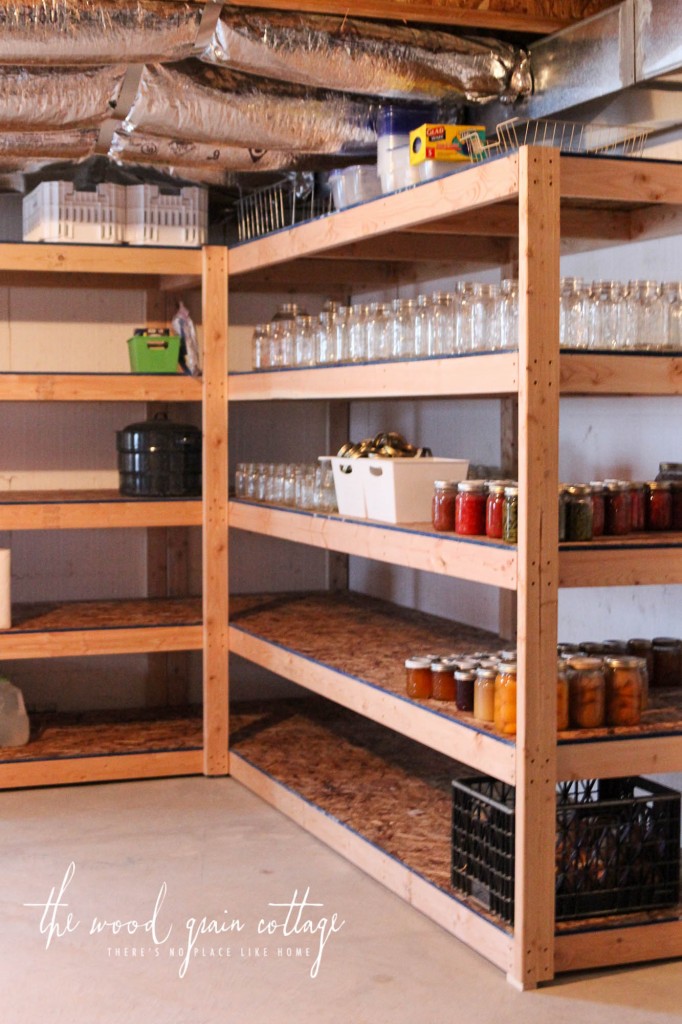This is a vertical color photograph of an open pantry situated in an unfinished room, possibly a basement, illuminated either by daylight or artificial light. The setting includes visible silver insulation and HVAC ductwork above the shelving, indicating an unfinished space. The simple wooden shelving structure consists of 2x4s with low-quality press wood shelves, arranged in five layers. 

On the left-hand side of the shelves, there is a green box and a black tin. On the right-hand side, from bottom to top, there is a black crate containing unknown objects. The second-bottom shelf holds a variety of canned goods, likely including peaches and assorted fruits. The third layer features additional canned items, potentially including peppers based on the visible colors—reds, oranges, and greens. The fourth shelf contains mostly empty glass jars and a white container filled with gold objects. The topmost shelf has various containers and more jars.

At the bottom left corner of the photograph, written text reads "The Natural Grain Cottage. There's no place like home." This detailed depiction highlights the pantry's functional yet unfinished aesthetic, possibly used for canning or as storage for emergency preparedness.